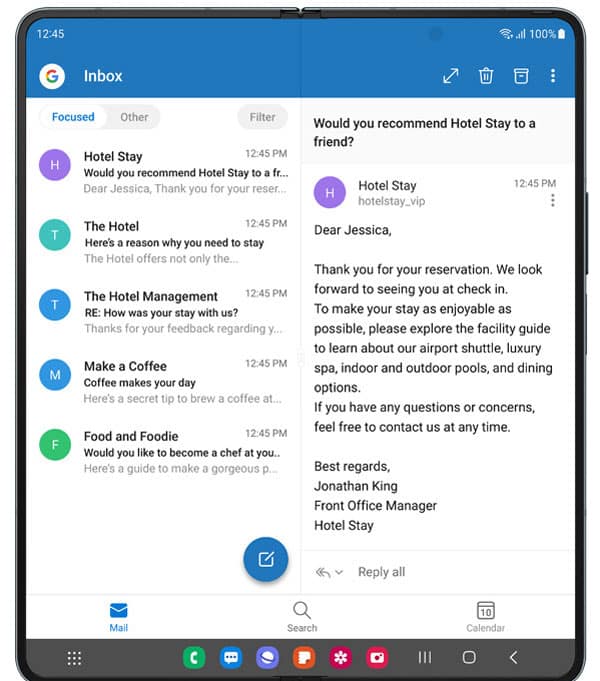The image showcases a modern, foldable Android phone, reflecting the latest trend in smartphone technology. The phone is unfolded, clearly displaying a subtle crease where the two halves meet. The screen exhibits an email application, likely a Google-based service, although it seems different from standard Gmail—possibly the discontinued Google Inbox app.

The visible inbox is filtered to highlight urgent or significant messages, as indicated by the "focused" tag. The emails predominantly pertain to hospitality and culinary topics. Subjects visible in the inbox include "Hotel Stay: Would You Recommend?", "Hotel: Here's a Reason Why You Need to Stay," "Hotel Management: How Was Your Stay With Us?", "Make a Coffee: Coffee Makes Your Day," and "Food: Would You Like to Become a Chef?" These messages suggest a potential influx of spam.

On the right side of the screen, one email titled "Would You Recommend a Hotel Stay to a Friend?" has been opened, potentially for further reading or action.